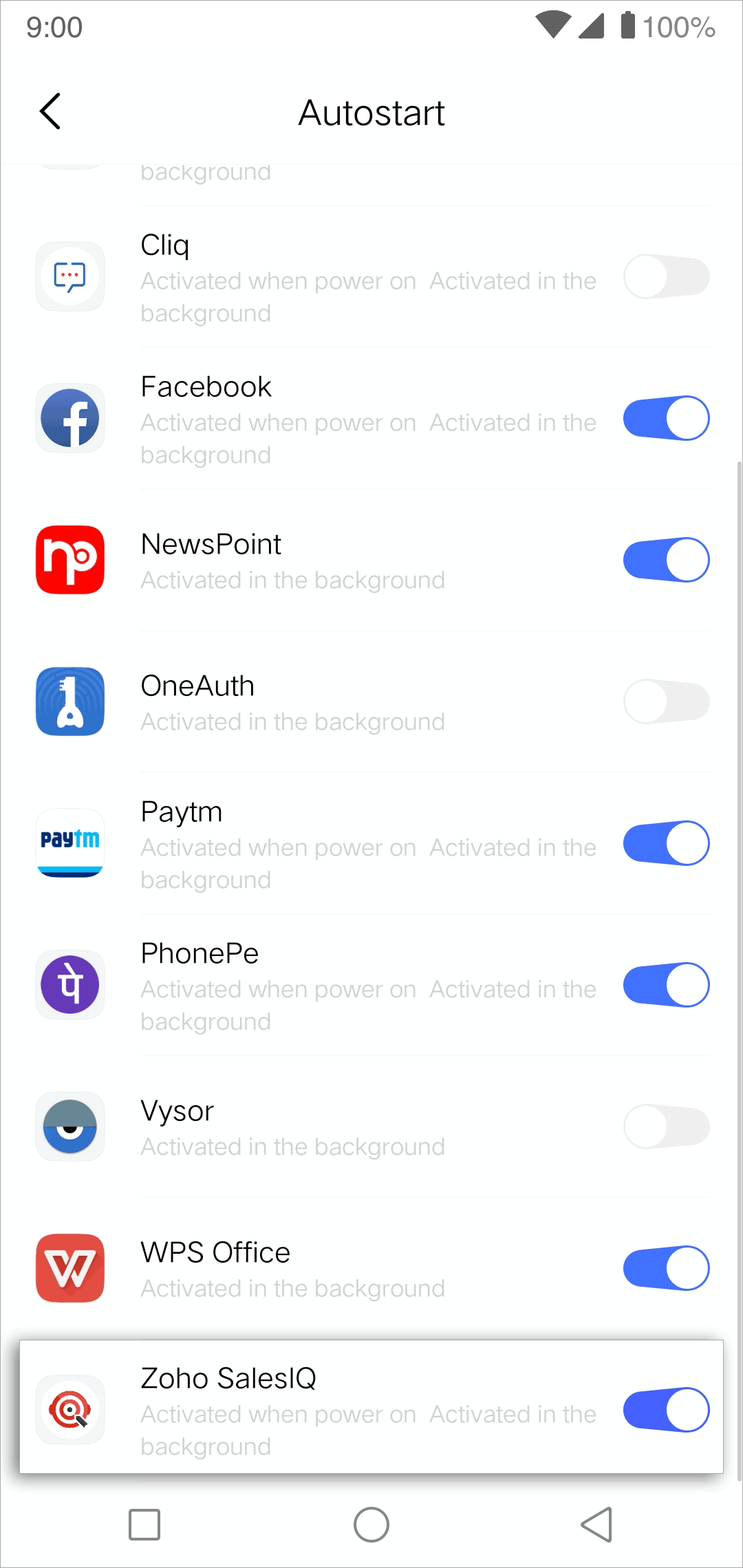The screenshot displays a phone settings interface under the "Auto Start" section. At the top of the screen, there is a back arrow on the left-hand side. Below this, the screen features nine app icons, each accompanied by a toggle button that either enables or disables the auto-start function for that app.

The apps and their respective toggle states are as follows:
1. Click - Off (gray toggle)
2. Facebook - On (blue toggle)
3. News Point - On (blue toggle)
4. One - Off (gray toggle)
5. KTM - On (blue toggle)
6. PhonePe - On (blue toggle)
7. Visor - Off (gray toggle)
8. WPS Office - On (blue toggle)
9. Zoho SalesIQ - On (blue toggle)

The background is predominantly white. Additionally, the top-left corner of the screen shows the time, which is 9:00, while the top-right corner displays the battery life at 100%.